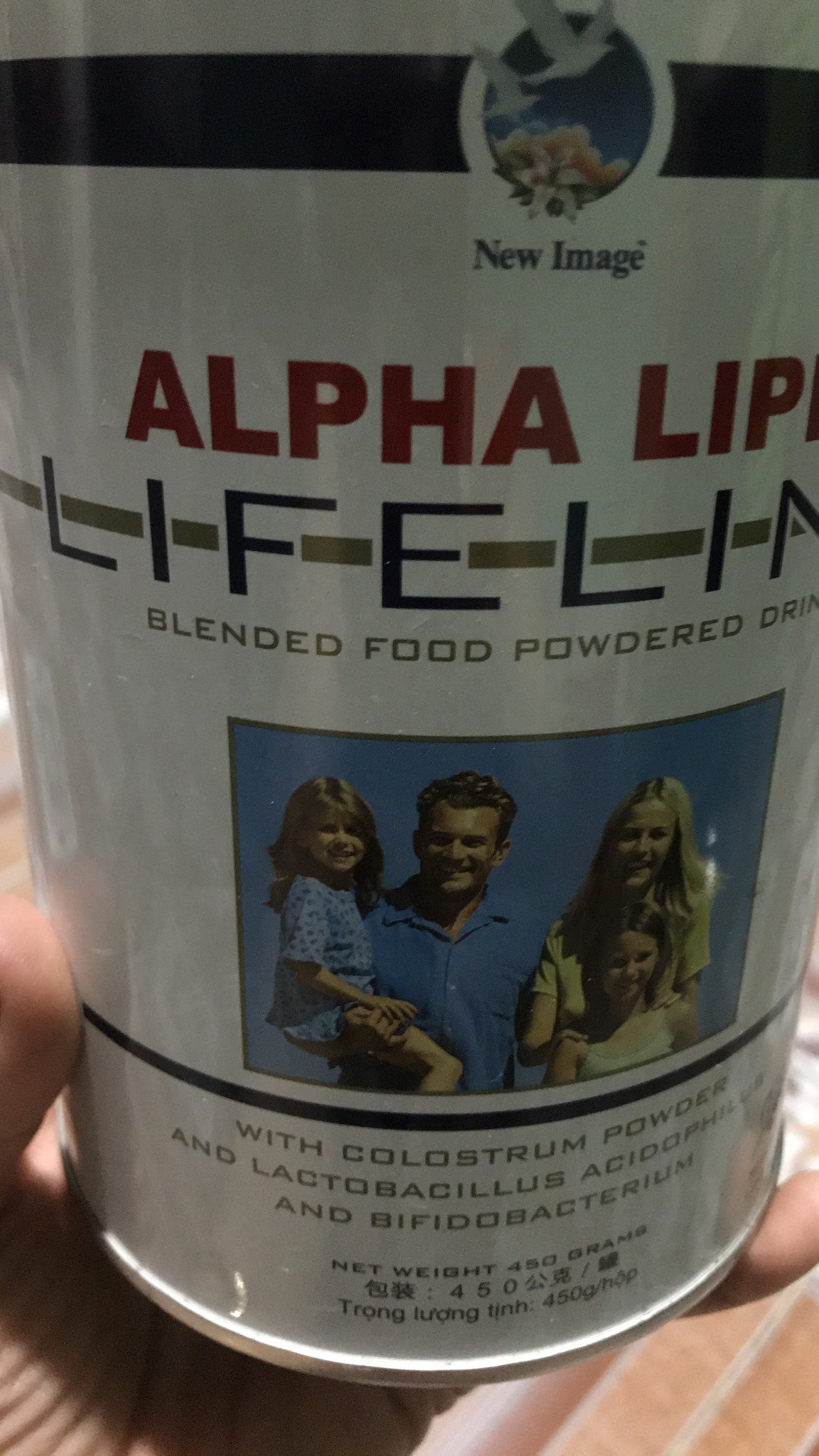**Descriptive Caption:**

The product appears to be from the brand "New Image," prominently displayed at the top of the can, accompanied by a circular logo featuring silhouettes of birds and flowers encased within a black-bordered band. The product name "Alpha Lip..." is partially visible, though it is heavily truncated, making the full name indiscernible. Similarly, the term "Lifeline" is also cut off. It is identified as a "Blended Food Powdered Drink."

The can's label features a family illustration: a man in a blue shirt holding a young girl, who is also dressed in blue. To their right stands a woman with blonde hair, her hands gently placed on the shoulders of the girl. Below this family portrait, the ingredients include "colostrum powder," "Lactobacillus acidophilus," and "Bifidobacterium." The product's weight is also listed on the can.

Encased in a shiny, white container, the can is highlighted against a rustic, brown stone surface, providing a warm, earthy contrast to the modern packaging.